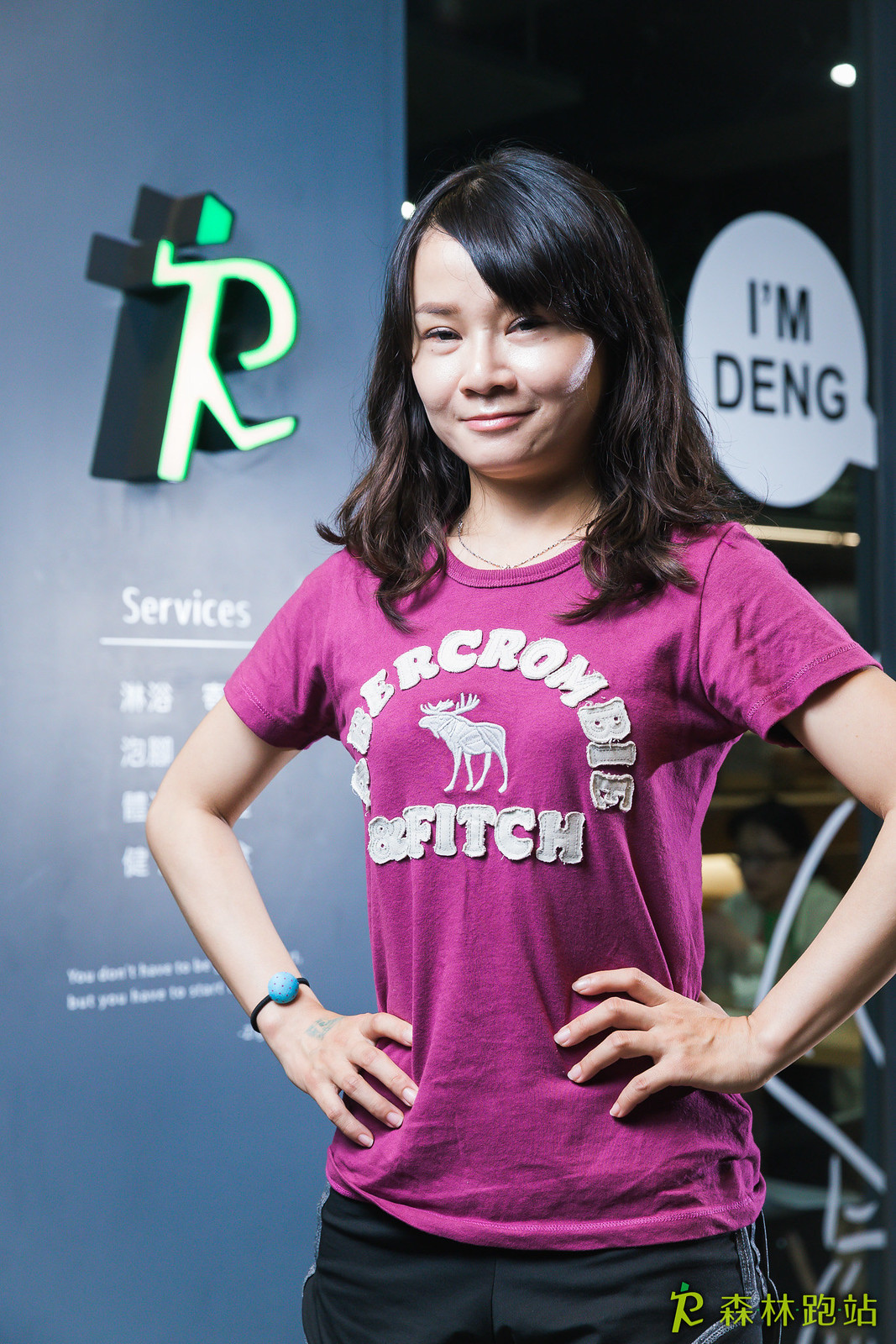The color photograph features a young woman, around 15 years old, standing confidently with her hands on her hips. She is looking at the camera with a slight smile, giving off an accomplished vibe. The woman has shoulder-length dark hair and Asian features, complemented by light brown skin. She's dressed in a purple Abercrombie & Fitch t-shirt adorned with white lettering and a moose in the center, paired with black pants. On her right wrist, she sports a bracelet that appears to be a hair tie with a blue ball.

Surrounding her are various elements adding context to the image. To the right, a seated figure with black hair and glasses can be seen, alongside a white speech bubble that reads "I'm Deng." On the left, a dark blue vertical banner displays a running stick figure logo at the top, followed by the word "Services" in white and some additional information likely in Mandarin. The bottom right corner also features foreign characters in yellow next to the same running person logo. The image's style leans towards photographic representationalism realism.